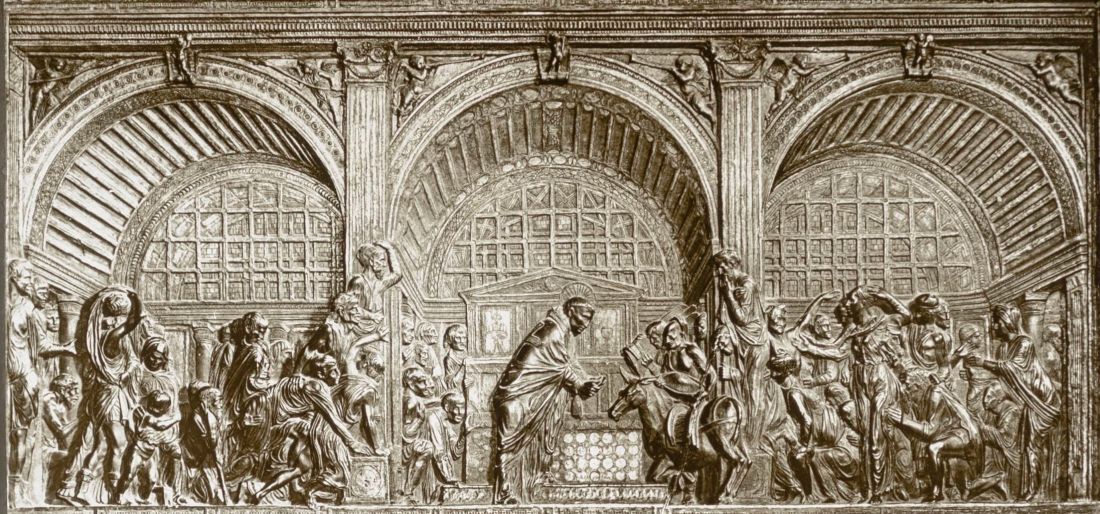The image portrays a panoramic relief sculpture, reminiscent of classical Roman or Renaissance art, featuring a lively scene rich with figures and detailed architectural elements. The artwork is symmetrically framed by three large, ornately coffered arches, which are supported by Corinthian columns and embellished with intricate designs, including images of individuals blowing horns and, on one arch, figures holding spears.

Underneath the arches, the scene is teeming with human figures dressed in ancient robes, engaged in a variety of activities. On the left side, a group appears to be in active discussion, with individuals carrying pots on their heads and climbing over objects, possibly a wall. There are also people who look like they're participating in rituals or focused conversations. In this panel, some figures are adorned with masks, adding an element of mystique and chaos.

The center of the composition is dominated by a man standing prominently in front of a podium, dressed in a toga-like garment. He appears to be the focal point, as numerous figures around him are directing their attention toward him, suggesting he may be delivering an important message or conducting a ritual. Nearby, a person on horseback, perhaps carrying wheat, interacts with a figure wearing a crown who is bending over a mysterious box, highlighting a moment of significance.

On the right-hand side, the scene mirrors some aspects of the left but is portrayed with more hectic energy. Here, individuals in robes are also climbing, carrying objects, and participating in what seems a more disorderly ritualistic gathering. The detailed arched ceilings above each segment beautifully encapsulate the narrative below, giving depth and grandeur to the scene.

Overall, the artwork is a monochromatic piece in shades of gray, suggesting an ancient artifact possibly etched in stone or metal. The meticulously engraved architectural features and the dense assembly of figures capture an old-world ambiance rich with historical and cultural significance, akin to works by masters like Michelangelo or Da Vinci.